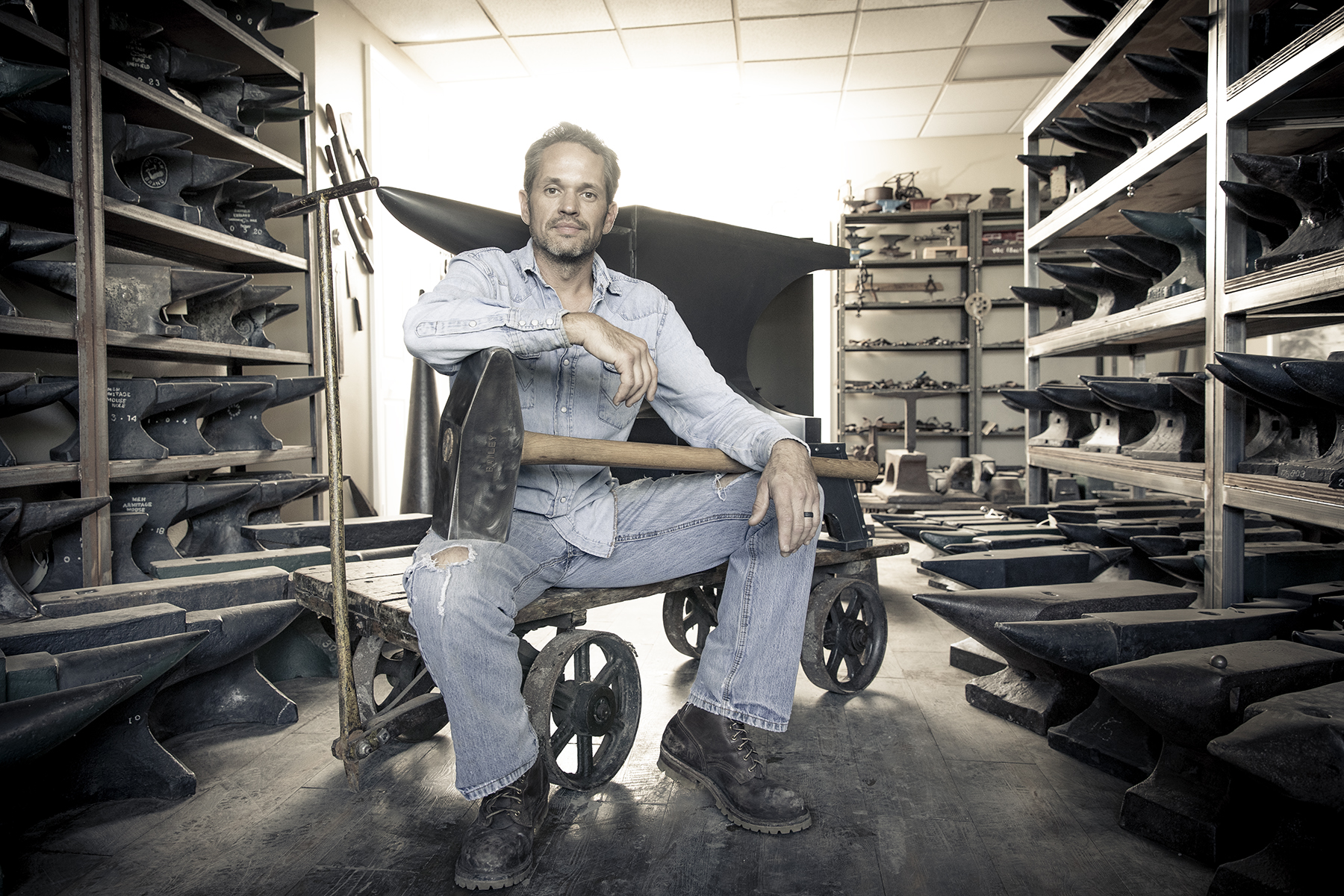In this detailed, horizontally-oriented photograph, we see a middle-aged man with medium skin and salt-and-pepper hair, sitting on an industrial wooden pallet cart with large steel wheels. He is dressed in a long-sleeve denim jacket, ripped denim jeans, and black work boots. The man appears to be holding a large sledgehammer, the iron head of which is black and marked, while the handle is brown. One of his arms is leaning on the hammer as it rests on his leg, and his other arm is also resting on the hammer's handle, suggesting the heft and weight of the tool. The setting seems to be a workshop or an anvil factory, evidenced by the numerous black anvils on wooden shelves to his left and right and even more anvils lining the floor. Behind him, there is a particularly large anvil positioned on the cart. Additional shelves filled with various tools, trinkets, and hats can be seen in the background. The room has a hardwood floor and a white tile ceiling with bright lighting overhead, adding to the industrial atmosphere. The man has a satisfied look on his face, suggesting pride and contentment with his craft.